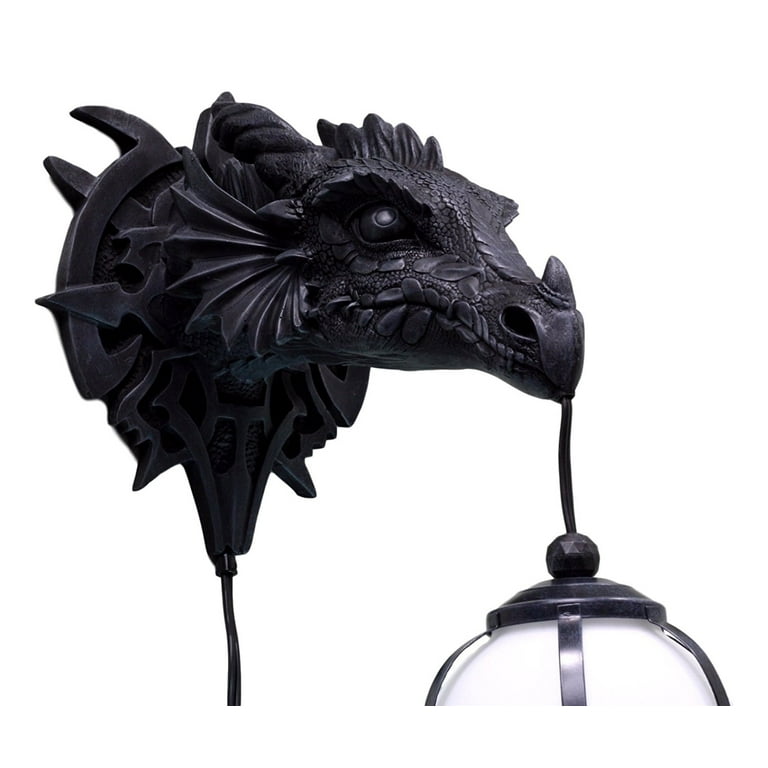This black and white photograph features a highly detailed wall sconce shaped like a dragon's head. The dragon, small and intricately carved with reptilian scales and other dragon-like features, has no visible ears but displays fin-like structures where its ears would be, and has a small horn on its nose. Additionally, it possesses a round crest with arrow designs protruding from the sides. The dragon's head is depicted in a monochrome black or dark gray die-cast metal, and appears to have glass eyes that catch and glint the light. 

The dragon is holding a round, white lamp globe with black accents in its closed mouth. The globe is fastened to the dragon's mouth by a short black cord that extends straight down. The dragon's head is mounted flush against the wall via an ornate, medieval-style backplate. An additional wire runs from the base of this backplate, presumably providing the necessary electricity to the light fixture. The fixture, which is reminiscent of an outdoor lamp, could be ideally suited for an entryway, contributing both practical lighting and elaborate, gothic decor.